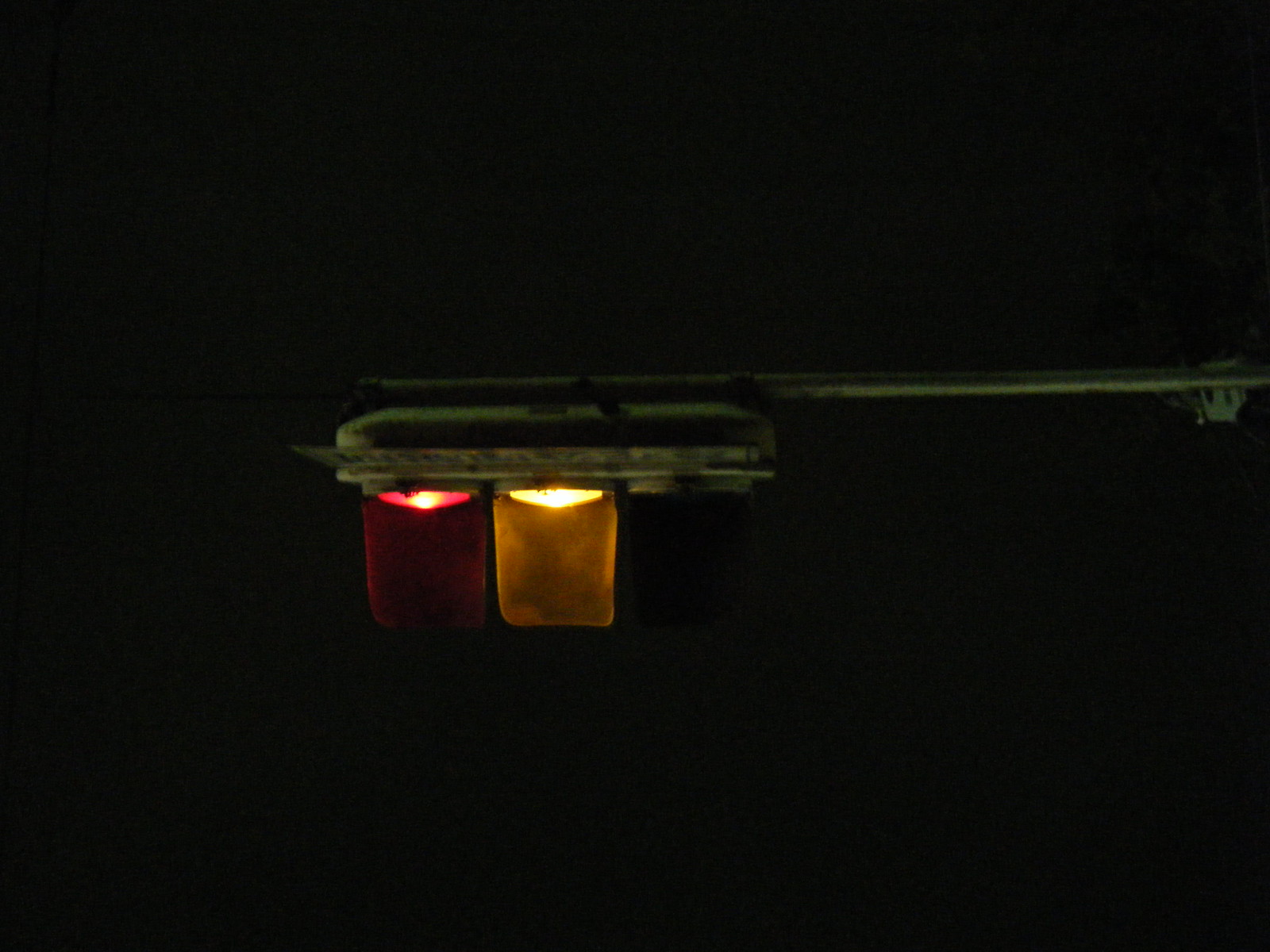The image features a nighttime, low-light photograph of what appears to be a traffic light captured from an unusual angle. The horizontal orientation of the photo reveals a silver, metal pole extending from the right side of the frame towards the center. Suspended from this pole, the traffic light displays illuminated red and yellow lights, while the green light remains unlit, making it difficult to discern in the darkness. The photograph is not only dimly lit but also slightly out of focus, adding to the challenge of identifying the scene with complete certainty.